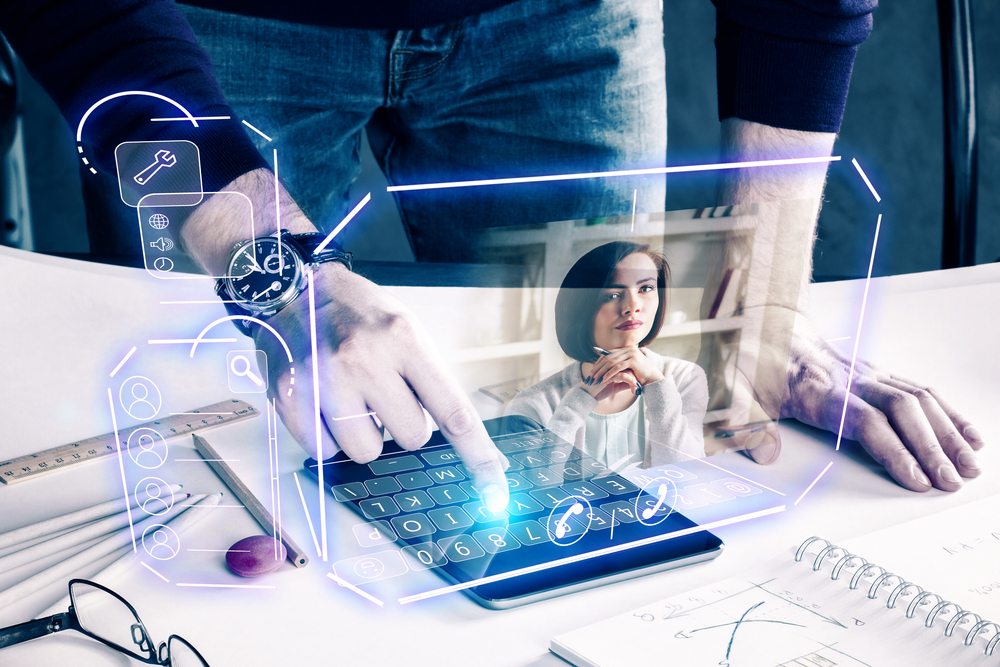In a futuristic office setting, a man is leaning over a sleek white desk, interacting with a small, advanced tablet positioned centrally. His left hand, flat on the desk, supports him while his right hand, adorned with a black watch, types on the tablet. The tablet, framed by a ruler, a pair of glasses, pencils, and a notebook, projects a holographic video conference screen. This screen displays a woman in a white sweater with her chin resting on her folded hands, holding a pen, and looking directly at the viewer. Her image seems to float above the tablet, emphasizing the cutting-edge nature of the technology. The man, only visible from mid-thigh down to his dark blue shirt and jeans, appears engaged in what could be a significant work-related call, potentially addressing either superiors or subordinates. Behind her, white bookshelves are partially visible, adding to the professional ambiance of the scene.